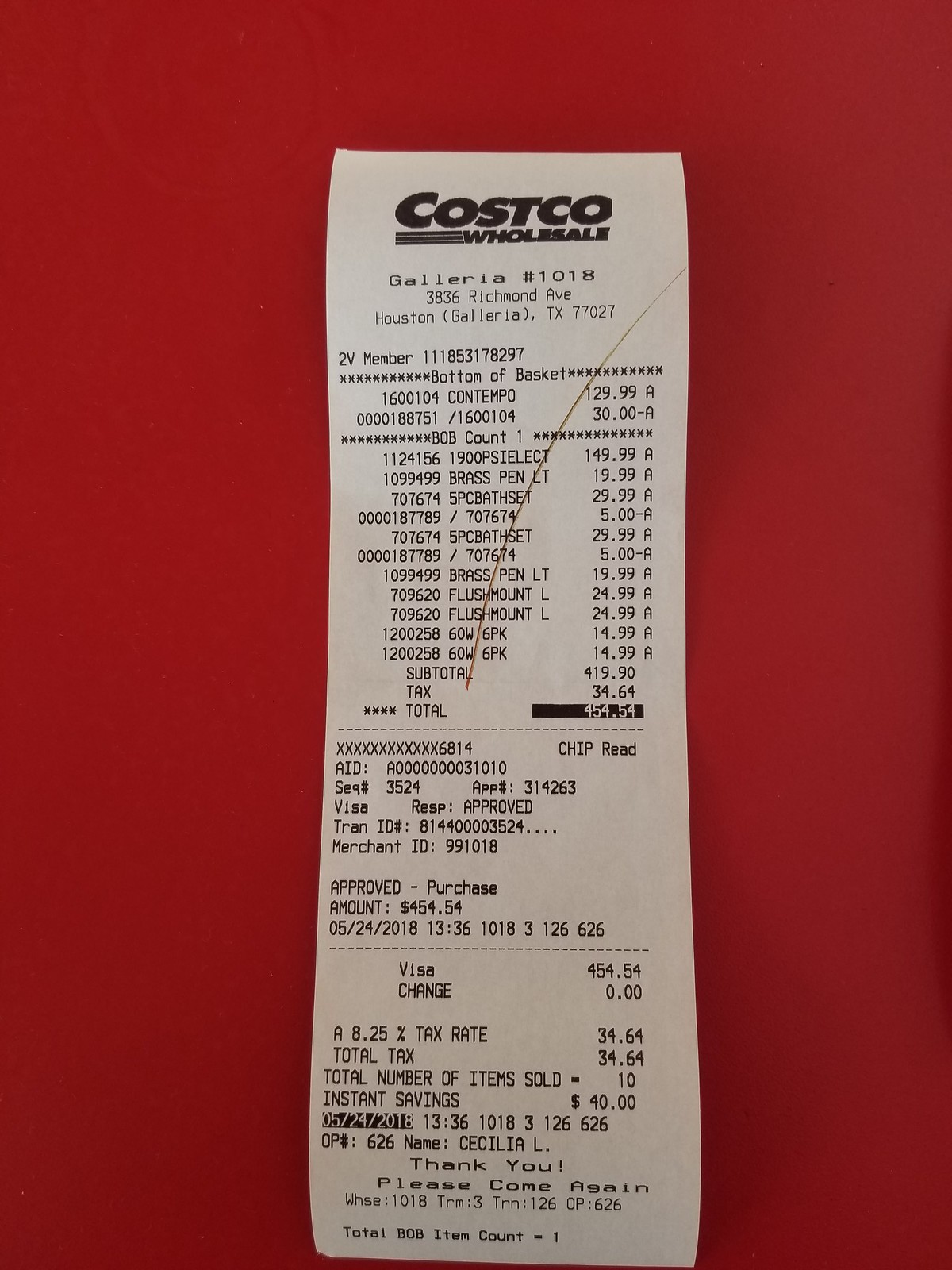A close-up photograph of a white receipt from Costco Wholesale is laid out on a vibrant red tabletop. The receipt features black lettering that includes the Costco Wholesale logo, followed by detailed store information: "Galleria number 1018-3836, Richmond Ave, Houston, (Galleria), Texas, 77027." The shopper's member number is visible, and the text "bottom of basket" appears, indicating examined items usually beneath the cart. The purchased items are listed meticulously, including a brass pen, a five-piece bath set (appearing twice), another brass pen, and two flush mounts. Additionally, a "B.O.B. count 1" is noted among the items. Below the list of products, payment information and the total cost including taxes are displayed. The bottom of the receipt reads, "Thank you, please come again." A red pen line is drawn through the products listed on the receipt, signifying that a Costco employee has checked the items.